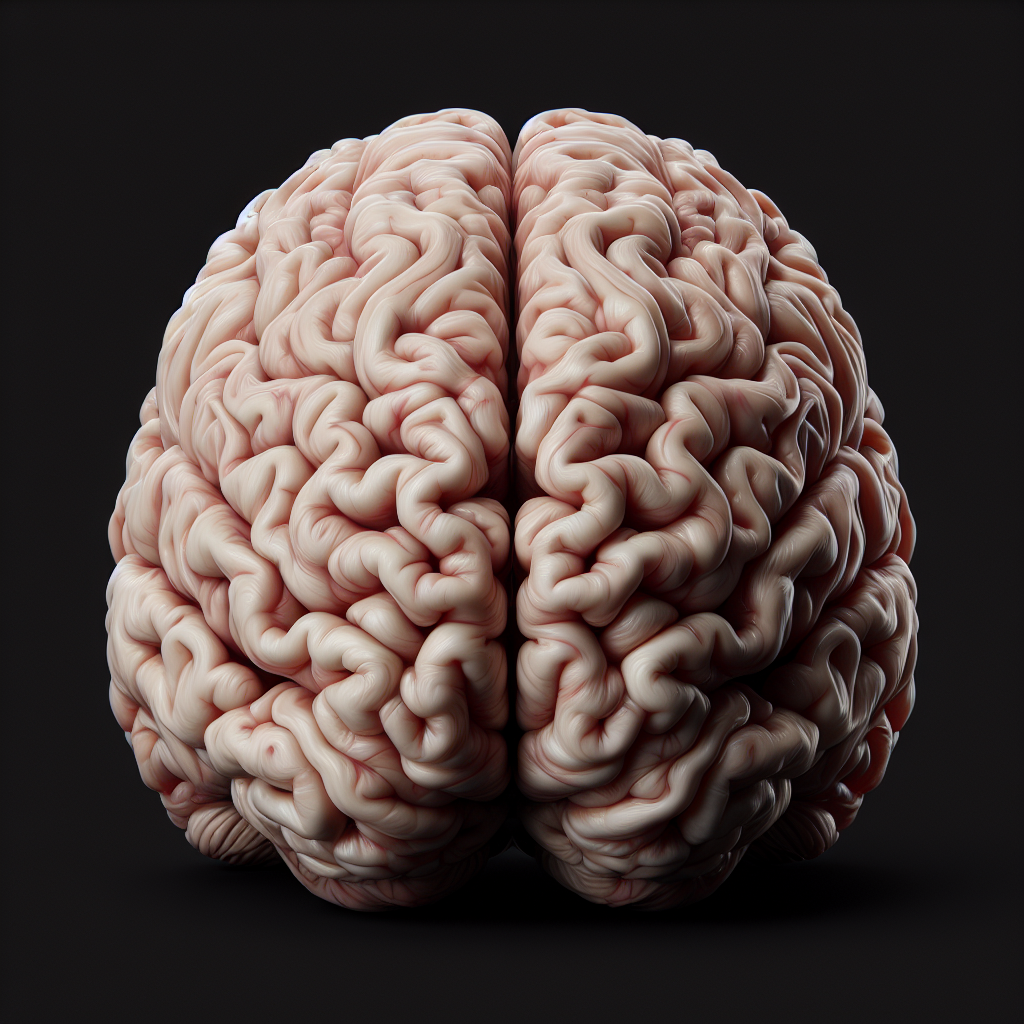The image depicts a close-up view of a human brain against a black backdrop. The brain, exhibiting a rounded and symmetrical structure, is split down the middle, with each half prominently displaying the intricate folds and curves characteristic of neural anatomy. The outer surface is marked by numerous knobby protrusions and interconnected fibers, appearing in a palette of pinkish, whitish, and grayish hues. The top portion of the brain is well-illuminated, highlighting the textured details and convolutions, while the bottom right side merges into shadow, creating a contrast with the light hitting the top. A shadow underneath the brain forms a V-shape, adding depth to the image. This depiction could either be an AI-generated graphic or a highly detailed plastic model of the human brain, given the lifelike yet potentially artificial features.